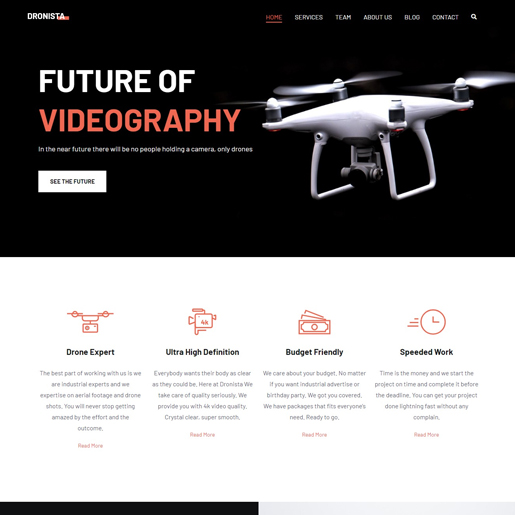The image depicts a screenshot of the homepage of a website titled "Dronista." At the top left corner of the page, the title "Dronista" is prominently displayed. On the top right, there are various navigation tabs arranged horizontally. The first tab, highlighted and underlined in orange, is labeled "Home." Subsequent tabs include "Services," "Team," "About Us," "Blog," and "Contact." Adjacent to these tabs is a magnifying glass icon, suggesting a search functionality.

Dominating the main portion of the page is a bold headline that reads "Future Videography." Below the headline, a subtext proclaims, "In the near future, there will be no people holding a camera, only drones." Beneath this statement is an inviting white button labeled "See the Future." To the right of the text, a sleek white drone is prominently featured.

Further down the page, several icons are neatly aligned, each with accompanying descriptions that presumably provide more information about various aspects of the website.